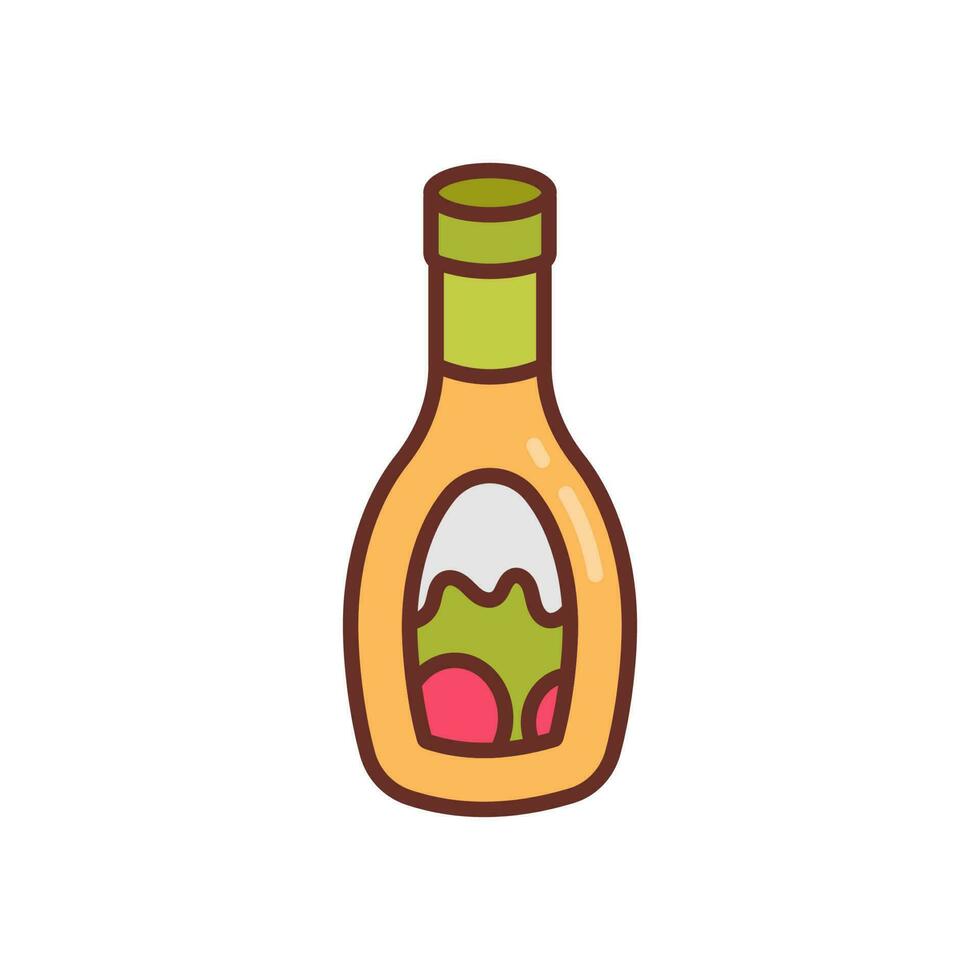This image features an animated, clip art-style illustration of a salad dressing bottle, resembling one filled with Thousand Island dressing. The bottle is primarily a light orange hue, topped with a contrasting green cap. The label adorning the bottle prominently displays graphics of a vibrant green lettuce leaf and two plump, red tomatoes. Among the illustrations, there's some white text in the background, though it is indecipherable. Encasing both the bottle and its label, a brown outline adds definition. The overall image is set against a stark white backdrop, providing no additional elements to gauge the bottle's scale.